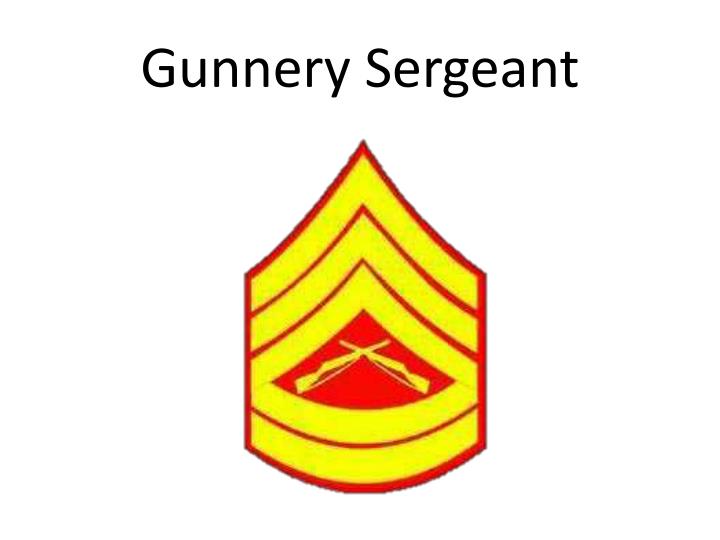The image features a gunnery sergeant emblem centered on a solid white background. At the top of the image, the words "Gunnery Sergeant" are written in black Arial font, with capitalized letters and slight spacing between them. Below the text, the emblem takes the form of a shield-like shape resembling a vertical rectangle with a rounded bottom that curves downward and a triangular point at the top. The emblem is outlined in dark red, with the interior featuring a yellow background. 

Within this yellow area, two prominent red zigzag lines and a solid red triangle are depicted. The red triangle is situated in the center and houses two yellow, diagonally crossed rifles with their barrels crossing over each other. Below these rifles are two curved, arched yellow stripes. The layering of shapes and colors creates the appearance of nested shields and highlights the intricate design elements of the emblem.